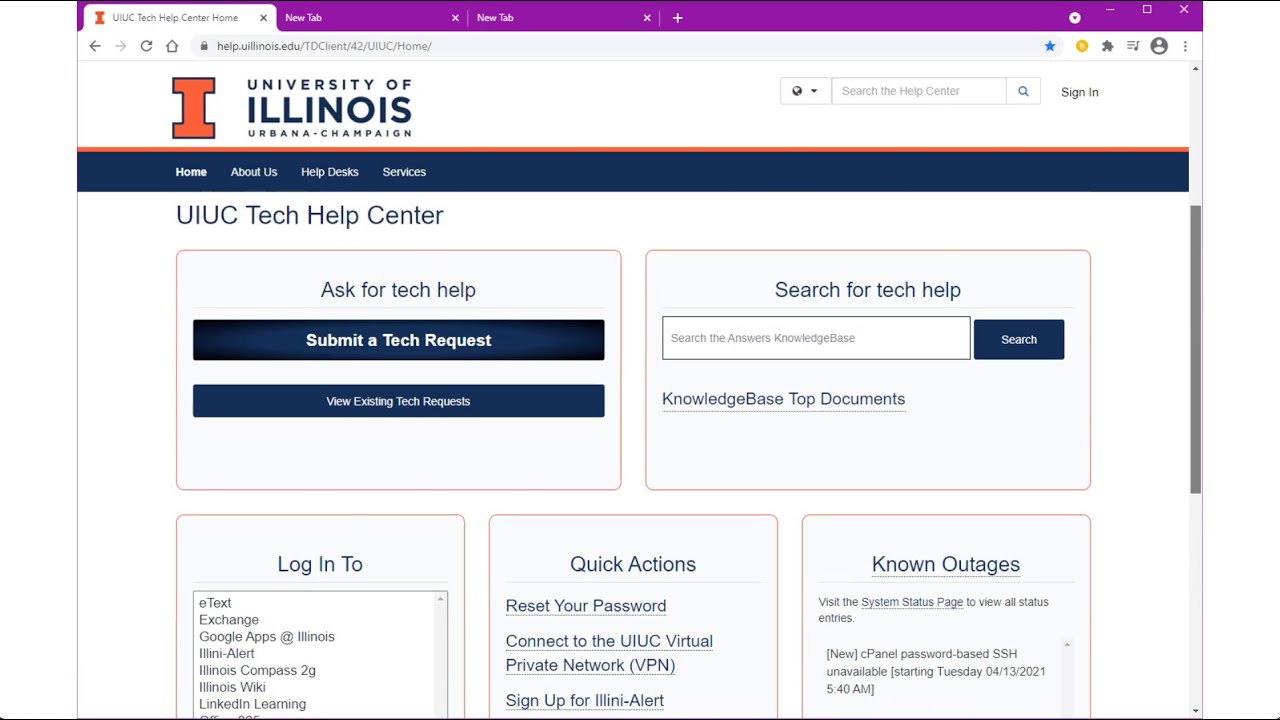The screenshot showcases the University of Illinois at Urbana-Champaign’s Tech Help Center webpage viewed in the Google Chrome browser. Two additional tabs are open in the browser, both labeled as "New Tab." The main tab features the Tech Help Center, where users can find various sections including "Ask for Tech Help," "Submit a Tech Request," and "View Existing Tech Requests." 

At the top right of the page, there is a comprehensive search bar that allows users to search the entire help center. Midway down the page on the right side, another search bar enables users to find specific tech-related assistance more easily. The layout is user-friendly, presumably designed by the university's IT department to streamline tech support for students and staff.

At the bottom of the page, there are several useful links and quick actions available, which include logging into different areas of the site such as email exchange, server access, and LinkedIn Learning. Additionally, quick actions like "Reset Your Password" are prominently featured to provide immediate assistance for common issues. The page is well-organized and clearly aims to facilitate easy access to tech support resources for the university community.